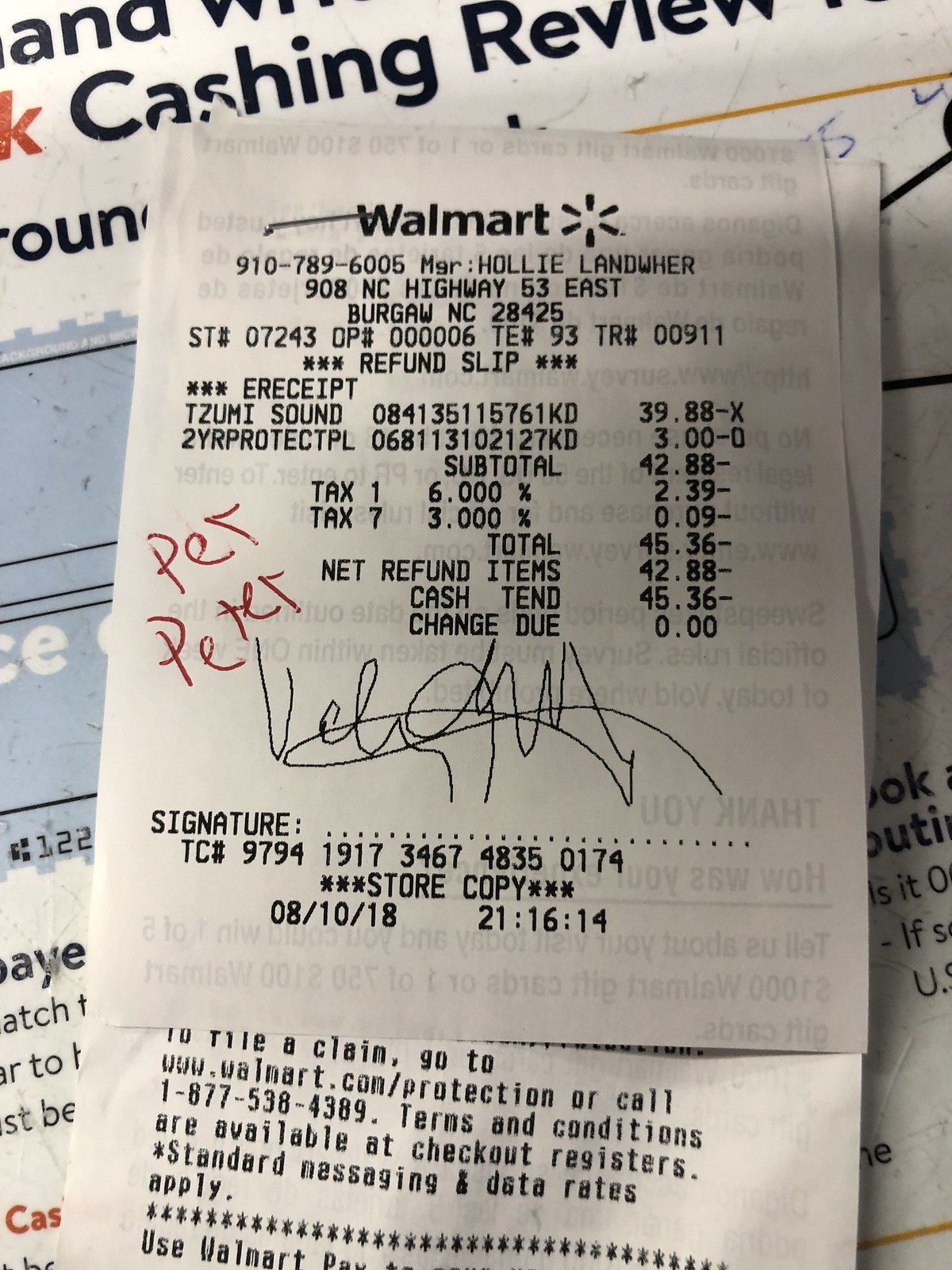The image features a Walmart refund receipt stapled to another receipt, placed on top of a light blue sample check that displays "Cashing Review" in black letters on a white background. The receipt, dated 08/10/18, is from the Walmart store located at 908 North Carolina Highway 53 East, Burgaw, North Carolina, 28425, managed by Holly Landwer. The receipt details the return of two items, priced $39.88 and $3.00, totaling $42.88. Including the tax and surcharge, the total is $45.36, with a notation stating "Cash Tendered $45.36, Change $0.00." There is a handwritten note in red ink reading "Per Peter" and a black signature, likely from the customer, completed on the store keypad.